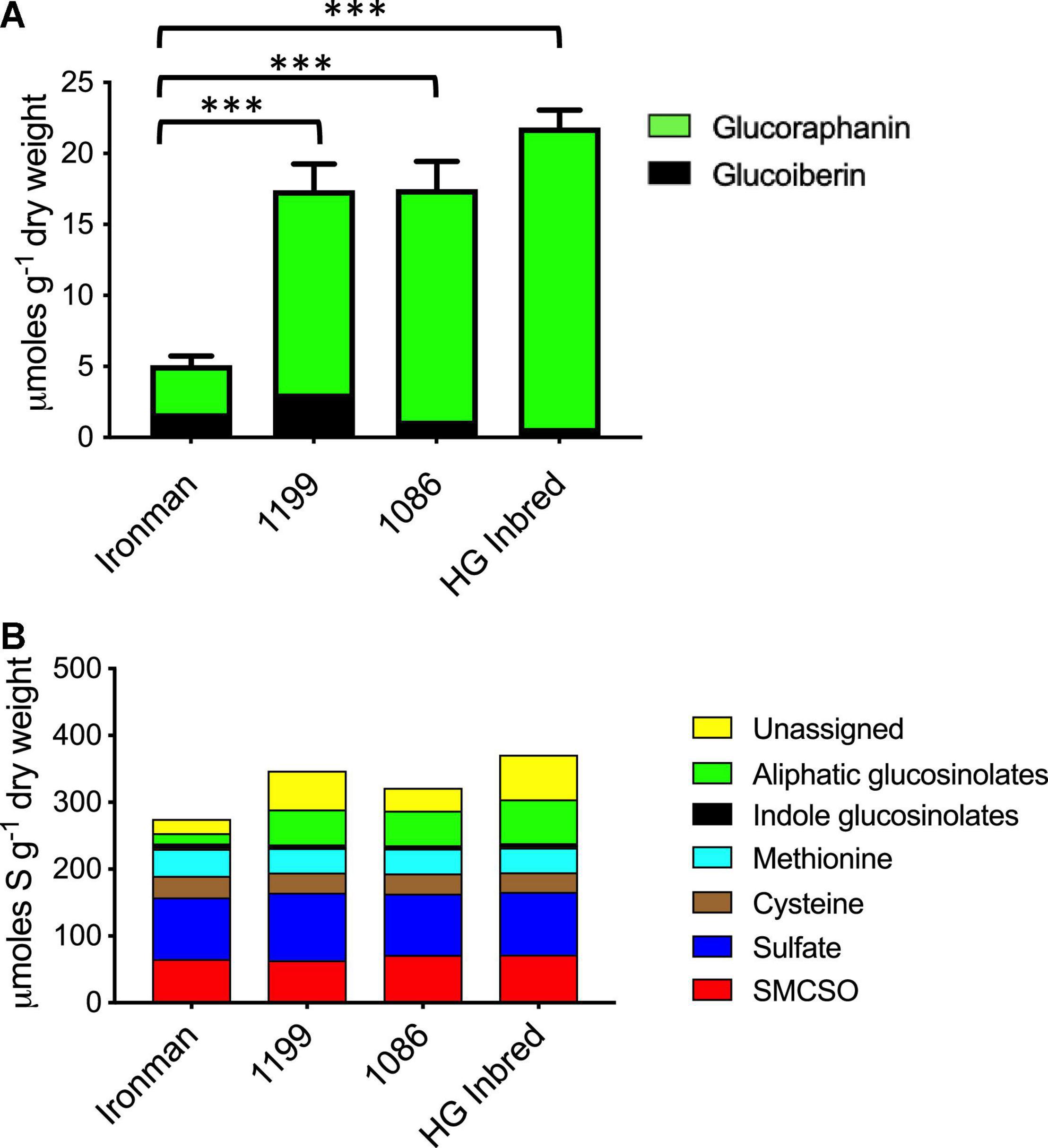The image features two detailed bar charts labeled A and B. Chart A, at the top, displays vertical bars in green and black representing the dry weight of M-O-L-E-S-G-1 moles. The vertical axis is marked with numerical values at intervals of 5, ranging from 0 to 25. The horizontal axis categorizes the bars under labels: Iron Man, 1199, 1086, and HG inbred. The categorized data shows Iron Man with a green and black bar extending slightly above 5, both 1199 and 1086 reaching just below 20, and HG inbred at around 20. Each bar has a T-shaped error bar on top, accompanied by a series of brackets and three asterisks beneath the chart. The color legend indicates that green represents glucoraphanin and black represents glucoibarin.

Chart B, positioned below, also measures dry weight but is noted as M-O-L-E-S-S-G-1. The vertical axis ranges from 100 to 500, marked in increments of 100. The horizontal axis retains the same categories: Iron Man, 1199, 1086, and HG inbred. In this chart, Iron Man is represented by a bar slightly below 300, 1199 by a bar around 350, 1086 by a bar near 375, and HG inbred by a bar just under 400. This chart uses a variety of colors for its bars: yellow for unassigned, green for aliphatic glucosinolates, light blue for methionine, brown for cysteine, blue for sulfate, and red for SM-CSO, as indicated in the legend on the right.